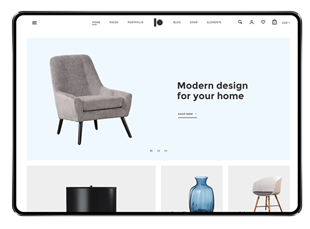Here is the refined and detailed caption for the image:

"This is a horizontally-oriented screenshot, likely from a tablet, displaying a website that appears to sell furniture. The rectangular screenshot is outlined in black with slightly rounded corners. Dominating the page is a large, horizontally extending light blue box. On the left-hand side of this box is an image of a gray-colored lounge chair or side chair. The chair is positioned with its back facing to the left, slightly leaning back at an angle. It features flat armrests on each side and outward-slanting wooden legs at each corner. To the right of the chair, the text 'Modern Design for Your Home' is prominently displayed."